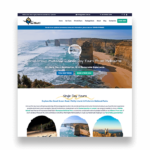This image showcases a website with a detailed layout. At the very top, there is a slim black rectangle extending from left to right across the page. Directly below it is a white rectangular section, followed by a navy blue rectangle.

Within the white section, there are seven clickable areas marked by plain black text. Additionally, there is a green box that serves as a clickable element.

Further down, the main content area features a picturesque scene of water, cliffs, and large rocks jutting out into the water, giving the impression of a beautiful and serene location. This area also contains some textual content related to an advertisement, with a blue clickable box and an adjacent green clickable box.

Continuing down the page, a squiggly yellow line is visible underlining a few words, followed by a paragraph of text. At the bottom of the page, there are three images aligned horizontally: one on the left, one in the center, and one on the right, completing the detailed layout of this webpage.